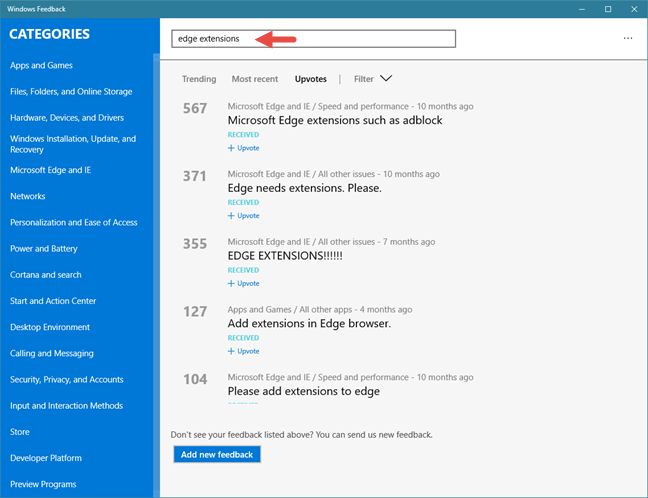The image displays a webpage dedicated to Windows Feedback. At the top, a teal banner prominently features the text "Windows Feedback," with both 'W' and 'F' capitalized. To the right of this banner are three icons: a dash, a square, and an 'X.'

On the left side of the page, a medium blue sidebar contains white text listing various feedback categories. These categories include:
- Apps and Games
- Files, Folders, and Online Storage
- Hardware, Devices, and Drivers
- Windows Installation, Update, and Recovery
- Microsoft Edge and IE
- Networks
- Personalization and Ease of Access
- Power and Battery
- Cortana and Search
- Start and Action Center
- Desktop Environment
- Calling and Messaging
- Security, Privacy, and Accounts
- Input and Direction Methods
- Store
- Developer Platform
- Preview Programs

In the center of the page, there is a search bar at the top labeled "Edge Extensions," accentuated by a red arrow pointing towards it. Below the search bar, the interface provides options to filter feedback by "Trending," "Most Recent," and "Upvotes" (with "Upvotes" in a darker text). Users can further refine results using a drop-down menu indicated by a down arrow next to "Filter."

Further down, the page lists Edge Extension feedback entries. At the very bottom, there is a prompt: "Don't see your feedback listed above? You can send us new feedback," followed by a button labeled "Add New Feedback."